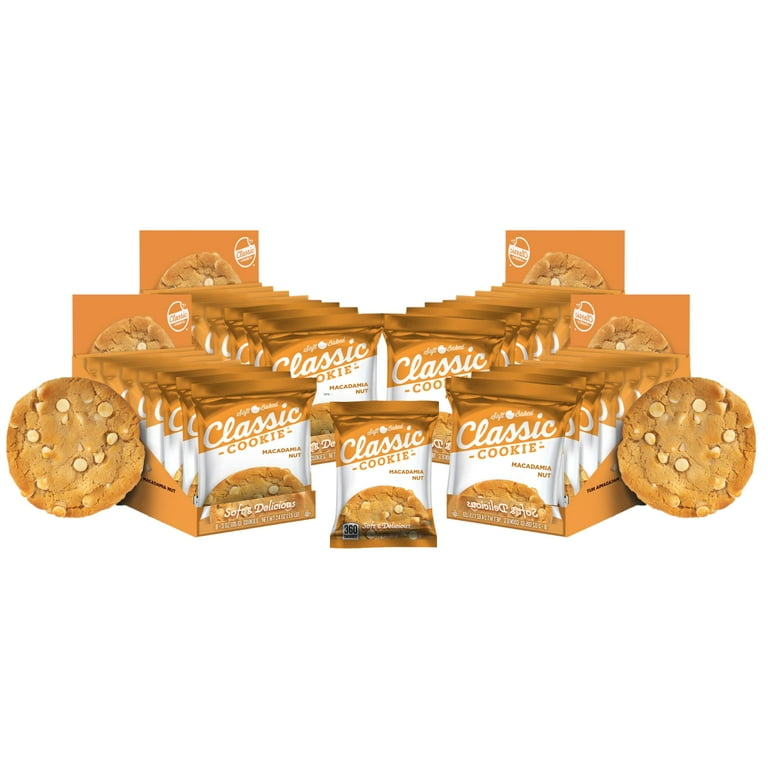This professionally staged image features a prominent display of individually packaged macadamia nut cookies by the brand "Classic Cookie." The packs, arranged in four distinct groups with one centered packet, are adorned in a white and gold color scheme, creating a visually appealing contrast. Each packet includes the brand name "Classic Cookie" written in white cursive, along with the flavor "Macadamia Nut" indicated below it. Adjacent to these packets on both the left and right sides of the image are two real cookies, light brown in color with visible macadamia nuts, providing a tangible representation of the product. A slogan at the bottom of the packaging reads "soft and delicious," and a small note signifies that each cookie contains 360 calories. The entire composition is set against a crisp white background, enhancing the clean and inviting presentation of these delectable, nutty treats.